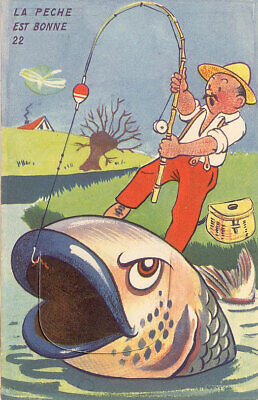The illustration is a detailed cartoon of a fisherman standing on a grassy riverbank, trying to catch an enormous, cartoonish fish with a fishing pole that is bent double under the strain. The man, depicted with a small black mustache, wears a yellow straw hat, a white shirt, and rust-colored pants. By his side on the grass is a fishing creel, traditionally used for holding fish. The fish he's hooked has angry eyes and resists being pulled out of the water, nearly overpowering the fisherman. In the background, across the river, stands a tree and the red roof of a house against a blue sky. The upper left corner of the image features the text "La pêche est bonne, 22" in black print, suggesting it might be a French comic painting, possibly from around 1922. The vibrant scene is rich with primary colors, emphasizing a whimsical yet detailed portrayal of the fishing adventure.